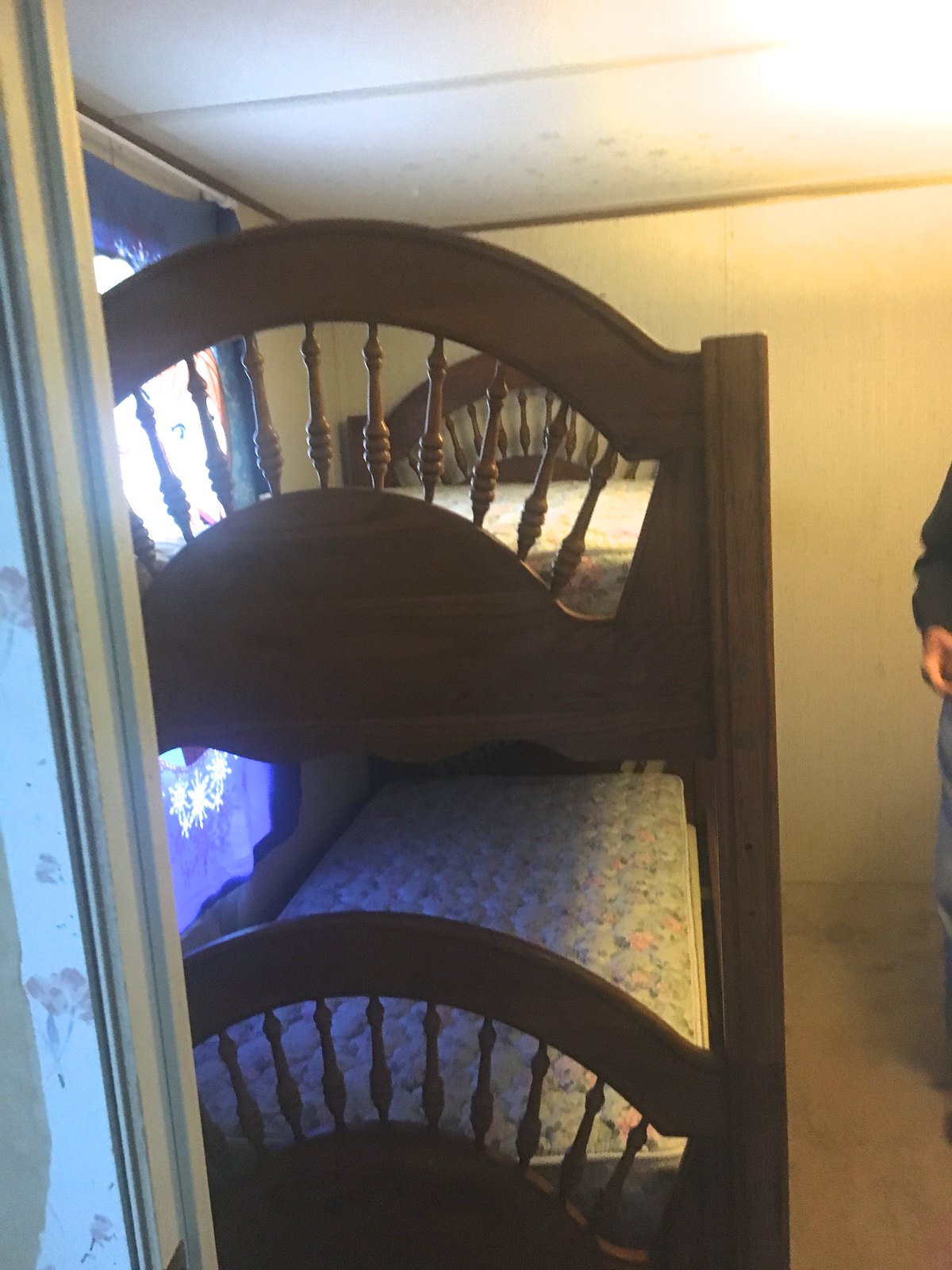The photograph depicts an antique-styled set of bunk beds inside a somewhat worn, aged bedroom. The image is taller than it is wide and is framed by a white doorway on the left. Beyond the doorway, against a tan wall aligned to the left side of the room, stand the bunk beds made of dark, handcrafted wood. The bed frames have an arcing, spoked design, reminiscent of old baby cribs, with intricate detailing on the headboards and footboards. Both the top and bottom beds reveal off-white mattresses adorned with a pink rose pattern. The floor below is likewise a tan color, adding to the room's muted palette. The overall ambiance of the room suggests wear and tear from extensive use. On the right side of the image, partially cut off, is the arm of a person, adding a subtle human element to the scene.